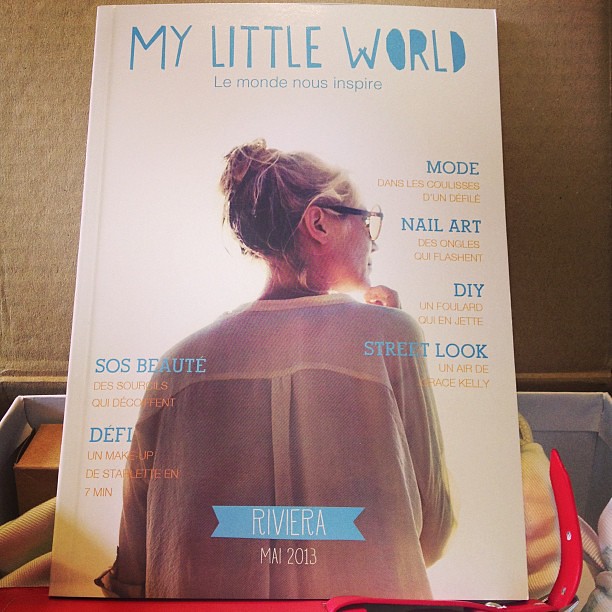This image is of a magazine or book cover featuring a white background. Dominating the top, in light blue capital letters, is the title "My Little World." Below that, the subtitle "Le Monde New Inspire" is written in French. The focal point of the cover is a photograph of a woman shown from the back, her image extending down to the bottom of the cover. She is wearing a long sleeve white button-up shirt, and her blonde hair is styled in a messy bun. The woman, who is Caucasian, is looking to her right, giving a view of her profile adorned with glasses. Her right hand is raised to her chin in a thoughtful pose.

On either side of the photograph is a series of headlines in blue and yellow text, primarily in French, including "Mode," "Nail Art," "DIY," "Street Look," "SOS Beauté," and "Défilé," each accompanied by additional text also in French. At the very bottom center of the cover is a ribbon-like label that reads "Riviera, Mai 2013."

The magazine or book is placed inside a gray basket, which also contains items in yellow and red colors. The background above and behind the basket features a cream-colored, textured wall.